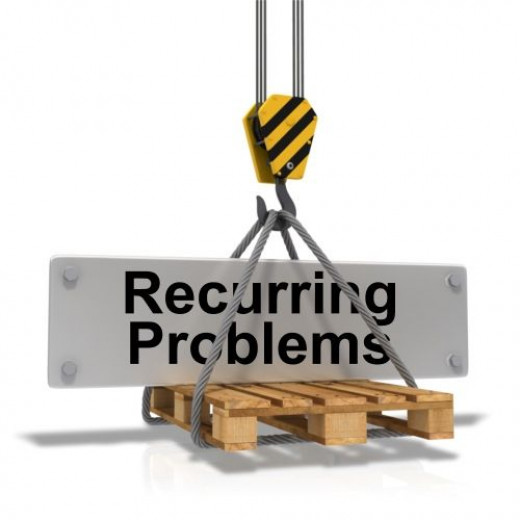The clip art image depicts a wooden pallet crate being lifted off the ground by a descending metallic gray hook. The hook is connected to three ropes that emanate from a black and yellow hexagon-patterned base, indicative of a crane's safety strap connection. The crate’s wooden slats are visibly nailed in place, typical of the kind used in warehouses for stacking goods. Secured atop the crate is a long, horizontal gray steel slab, bolted on the top and bottom. Bold black text on the slab reads "Recurring Problems". The background of the image is a stark, plain white, further emphasizing the clip art style of this clearly illustrated, non-realistic scene.